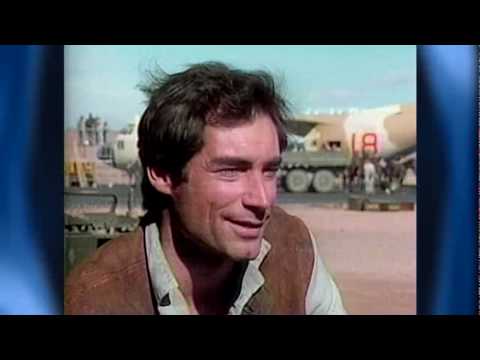The image appears to be a still from a movie or TV show, possibly featuring James Bond, specifically Timothy Dalton. In the foreground, a light-skinned man with brown hair—dressed in a tan or light brown vest over a white or cream-colored shirt—is the primary focus. He stands on what appears to be an airstrip, positioned sideways and looking off-camera with a smile. The background includes an old military plane in brown and tan colors, marked with the number "L8" in red lettering, as well as an army Humvee and blurred figures who seem to be working on the plane. The scene is framed by blue bars on the sides, suggesting it may be a vintage or stylized shot, contributing to an overall war-time or historical context. However, the man’s relaxed demeanor introduces a contrast to the otherwise tense ambiance.